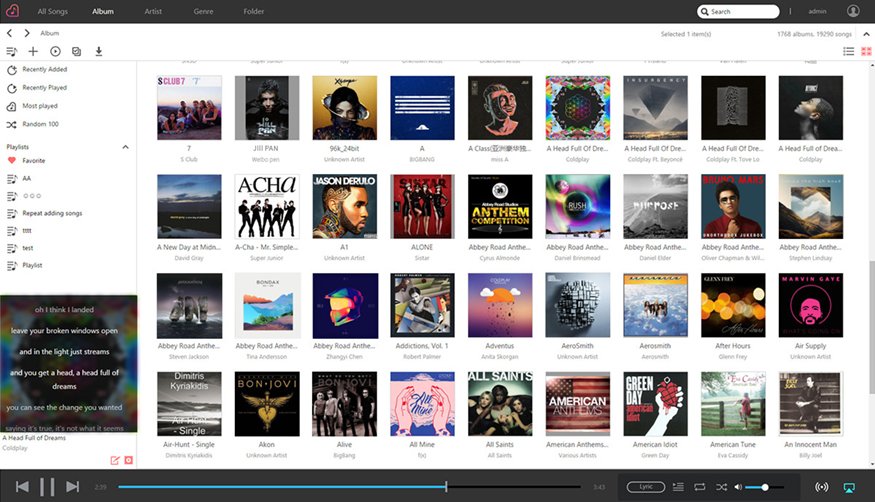This image depicts a detailed interface of an audio streaming website. At the top left, there's a distinctive orange heart logo, tilted on its side. Adjacent to the logo are several navigation categories: "All Songs," "Album," "Artist," "Genre," and "Folder."

On the top right, the image shows a user's profile section containing a circular profile picture and a username that starts with the letter "A" (the remainder is too small to decipher). To the left of the profile section is a search bar for easy access to the website's content.

The central portion of the interface displays an array of album covers. There are four rows in total, each containing nine categories, showcasing a wide range of music.

On the far left, directly beneath the navigation categories, there are additional sections labeled: "Recently Added," "Recently Played," "Mint List," and "Random Song." Below these sections are options for "Playlist" and "Favorite," with a red heart icon beside the "Favorite" option. Further down, there are placeholders or categories labeled with cryptic titles such as "Double A," "Circle, Circle, Circle," "Repeat Adding Songs," and "Playlist Test."

At the very bottom left, in a distinct square area, there's an album cover featuring lyrics in white text overlaying the image.